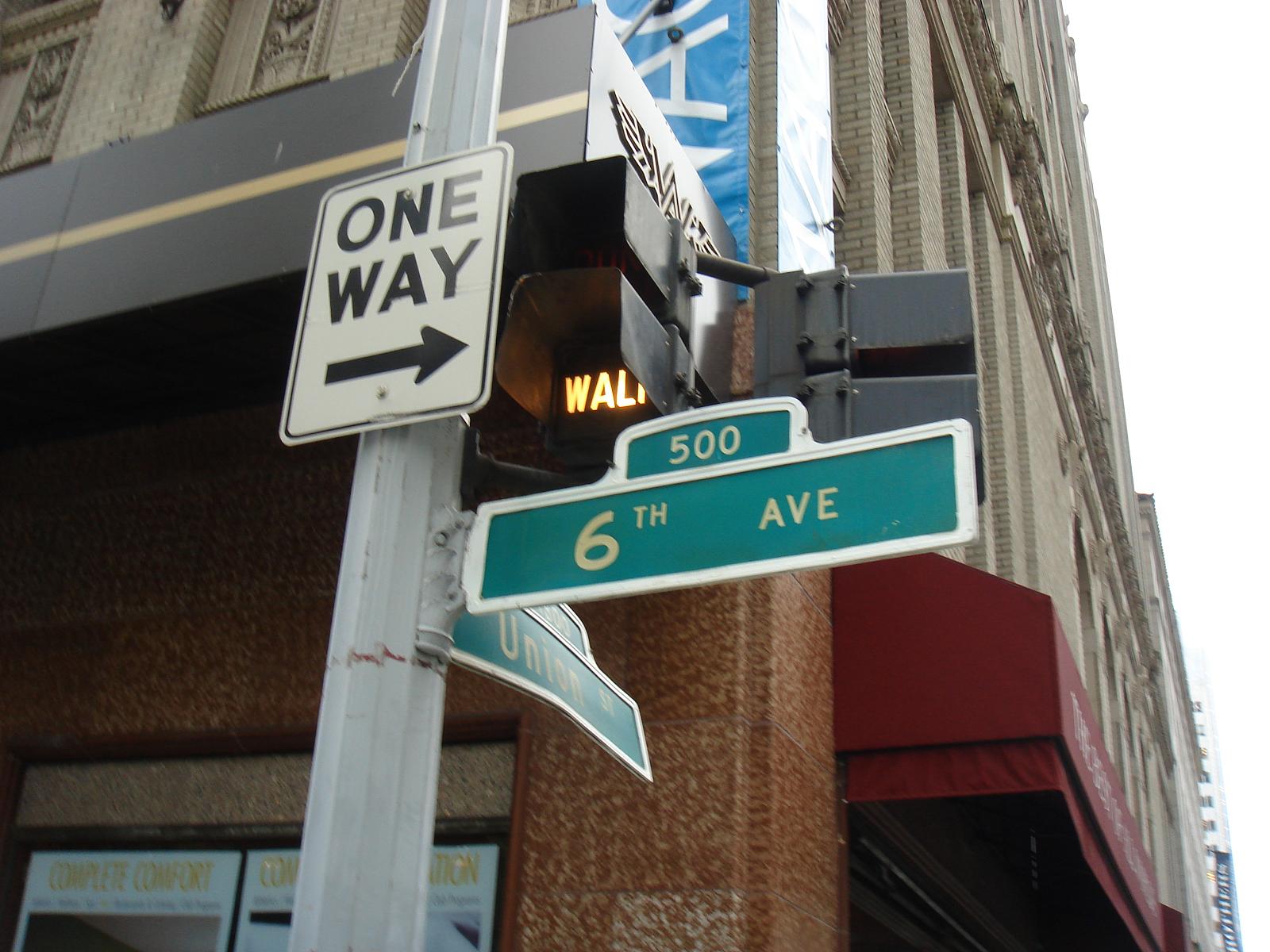This image captures a close-up view of an urban street corner. Dominating the left side of the frame, a vertical silver pole with divoted edges supports multiple street signs and pedestrian signals. Mounted prominently at the top of the pole is a white rectangular one-way sign with black letters and a black arrow pointing to the left. Below and to the right, a green street sign displays "6th Ave" alongside the block number "500" in a smaller, curved silver frame. A perpendicular sign reading "Union Street" is visible, though its block number is obscured. Directly beneath these street signs, a pedestrian signal shows an illuminated white walk symbol. The camera captures a tall urban building with ornate beige-tan brickwork and intricate relief carvings in the background, along with a notable red awning extending towards the side, suggesting a possible government building or cultural institution.